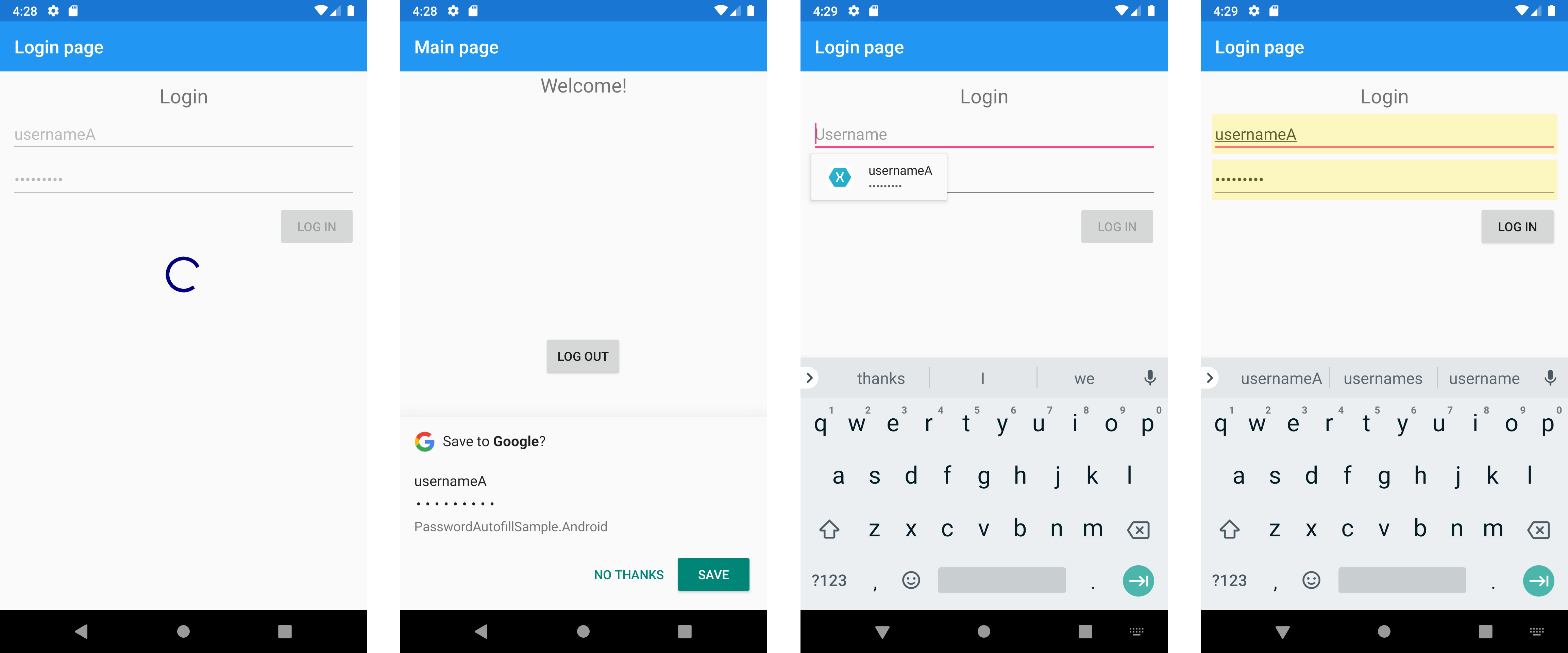**Detailed Caption:**

The image consists of four vertically aligned rectangular screenshots, each depicting different stages of a login process. 

1. **First Screenshot (Far Left):** This is the initial login page, featuring a simple interface. The heading reads "Login" in bold black text. Below this, there is a field labeled "Username" with an entry placeholder "A." Underneath the username field, there is another field with several dots representing a hidden password. At the bottom of the form, a button labeled "Login" can be seen. Additionally, there is a three-quarter open, three-quarter closed circle icon present, possibly indicating an option for password visibility.

2. **Second Screenshot (Second from Left):** This screenshot displays what appears to be the main page of the application, which has a white background. At the top, it says "Main Page" in white text, followed by a greeting "Welcome" in gray text. At the bottom of the page, there's a "Logout" button available. Below this, there's a prompt for saving login details to Google, which shows "Username: A" and a hidden password represented by a series of dots. The screen includes options with "No thanks" in plain text and a highlighted "Save" button.

3. **Third Screenshot (Second from Right):** This image shows another iteration of the login page. The header again reads "Login" in gray text. Below this, there is a username field where a pop-up appears, showing the username that was saved to Google. Beneath the username entry, the "Login" button is present but not highlighted. The bottom portion of the screenshot shows an on-screen keyboard from a cell phone, indicating that text input is active.

4. **Fourth Screenshot (Far Right):** This screenshot is also of the login page with a white background. The header reads "Login" in gray text. The username field displays "Username: A," which is highlighted in orange or yellow. Below this, the password entry field shows a series of dots, also highlighted in yellow. The "Login" button is visible underneath these fields. At the bottom of the screen, the cell phone's keyboard is partially shown, indicating text input functionality.

Overall, the sequence of screenshots details the user interface flow from logging in to saving credentials and revisiting the login page with autofill options.